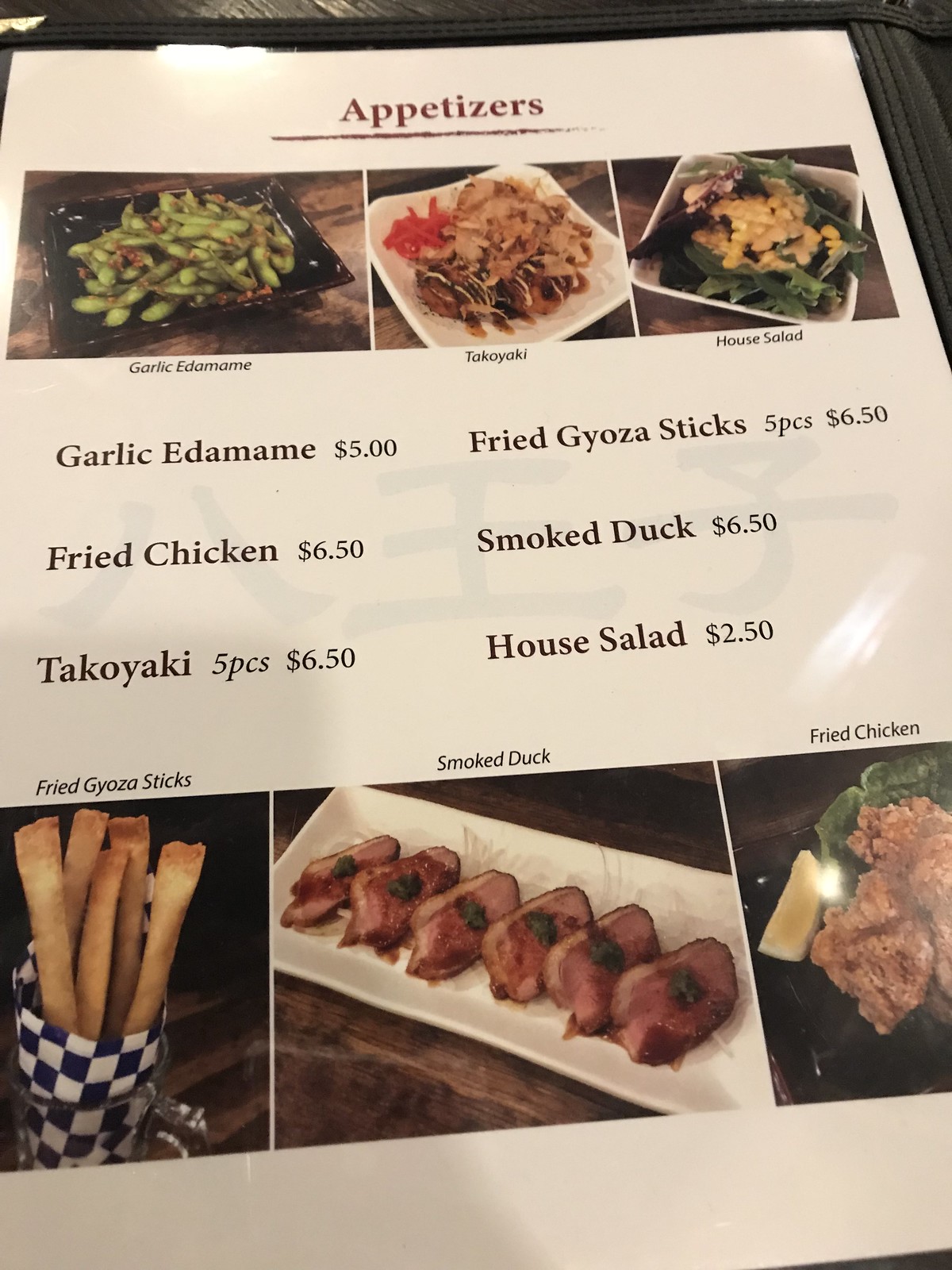This photo captures a section of a restaurant menu, specifically showcasing appetizers. Dominating the top portion of the menu are the words "Appetizers" prominently displayed. Beneath this heading, three images of various plated dishes are arranged horizontally, offering a visual preview of some of the menu options.

The lower portion of the menu lists six appetizer items, each accompanied by their respective prices. The items are as follows:

1. Garlic Edamame - $5
2. Fried Chicken - $6.50
3. Takoyaki (5 pieces) - $6.50

On the right-hand side, continuing from top to bottom, the additional appetizers include:

4. Fried Goya Sticks (5 pieces) - $6.50
5. Smoked Duck - $6.50
6. House Salad - $2.50

Below this list, three more images of the menu items are arranged in a similar fashion to those at the top. However, these images are not clearly visible in the photo.